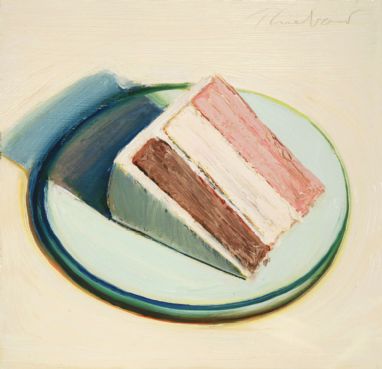The image is a realistic painting depicting a slice of ice cream cake placed on a white plate with a blue rim. The cake features three layers: a chocolate layer on top, a vanilla layer in the middle, and a strawberry layer at the bottom, all separated by white icing. Additional icing decorates the top of the cake slice. The cake is lying on its side, casting a shadow to the left, indicating the light source is from the right. The background of the painting transitions from tan to light pink. In the upper right corner, there is a faint, barely discernible artist's signature, possibly starting with a "T" and followed by an "H." There are no other elements or text in the image.